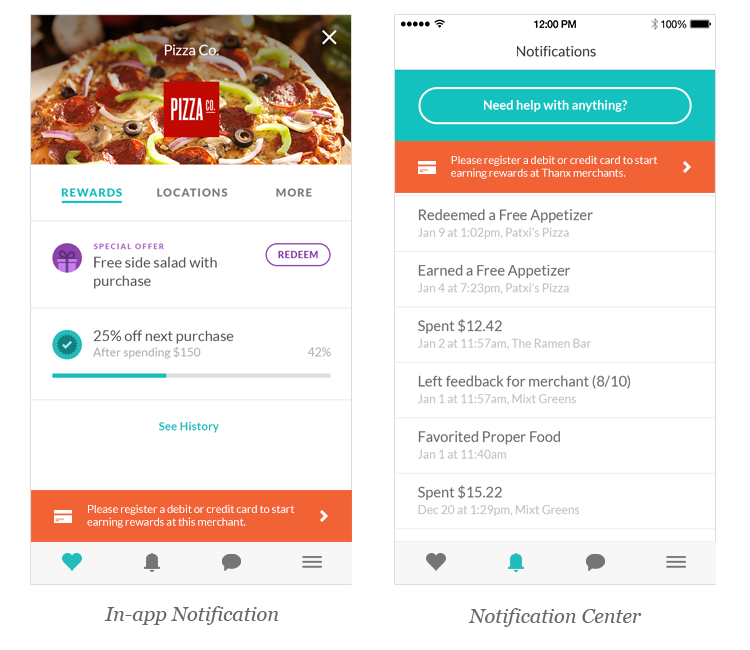The image consists of two tall, rectangular smartphone screenshots displayed side-by-side horizontally. The left screenshot features an in-app notification from "Pizza Company" and depicts the upper part of a mouthwatering pizza in a semi-circular shape at the top. Across the pizza image, the text "Pizza Company" is prominently displayed, with a matching red square in the center also labeled "Pizza Company".

Beneath the image, several lines indicate various sections such as Rewards, Locations, More, Special Offer, and the specific promotion "Free Side Salad with Purchase." Adjacent to these sections is an oval-shaped button labeled "Redeem." Below, there's an offer: "25% off next purchase after spending $150," accompanied by a progress bar that shows 42% completion towards this goal. At the bottom of the screenshot, it prompts users to "See History" and encourages them to "Please register a debit or credit card to start earning rewards at this merchant."

The right screenshot captures the Notification Center with the header "Notifications." Below it are several entries detailing user activities and transactions: "Need Help With Anything," "Redeemed a Free Appetizer," "Earned a Free Appetizer," "Spent $12.42," "Left Feedback for Merchant," "Favorited Proper Food," and "Spent $15.22." The Notification Center neatly lists these interactions, providing a clear and organized summary of the user's recent activity.